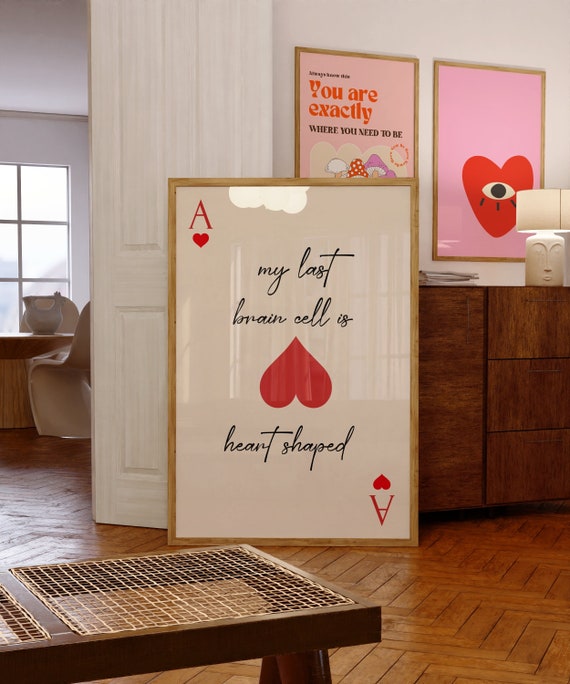The image depicts a cozy room, possibly a dentist's office or someone's home, characterized by a distinctly warm and welcoming ambiance. At the center of the composition is a large framed graphic design poster, resembling a playing card—the Ace of Hearts. The card, with its light wood frame and white background, prominently displays the text "My last brain cell is heart-shaped" above and below an upside-down red heart in the middle. Surrounding this are two other framed posters on the wall, one of which carries the motivational message, "You are exactly where you need to be," and another featuring the famous corporate heart symbol with an eye in the center. The setting includes a desk supporting a face-shaped lamp, paneled flooring in a dark brown wood finish, and an open door revealing an adjacent room with a window, table, and chairs in the background. The overall decor suggests a blend of professional and personal elements, creating a space that is both functional and inviting.